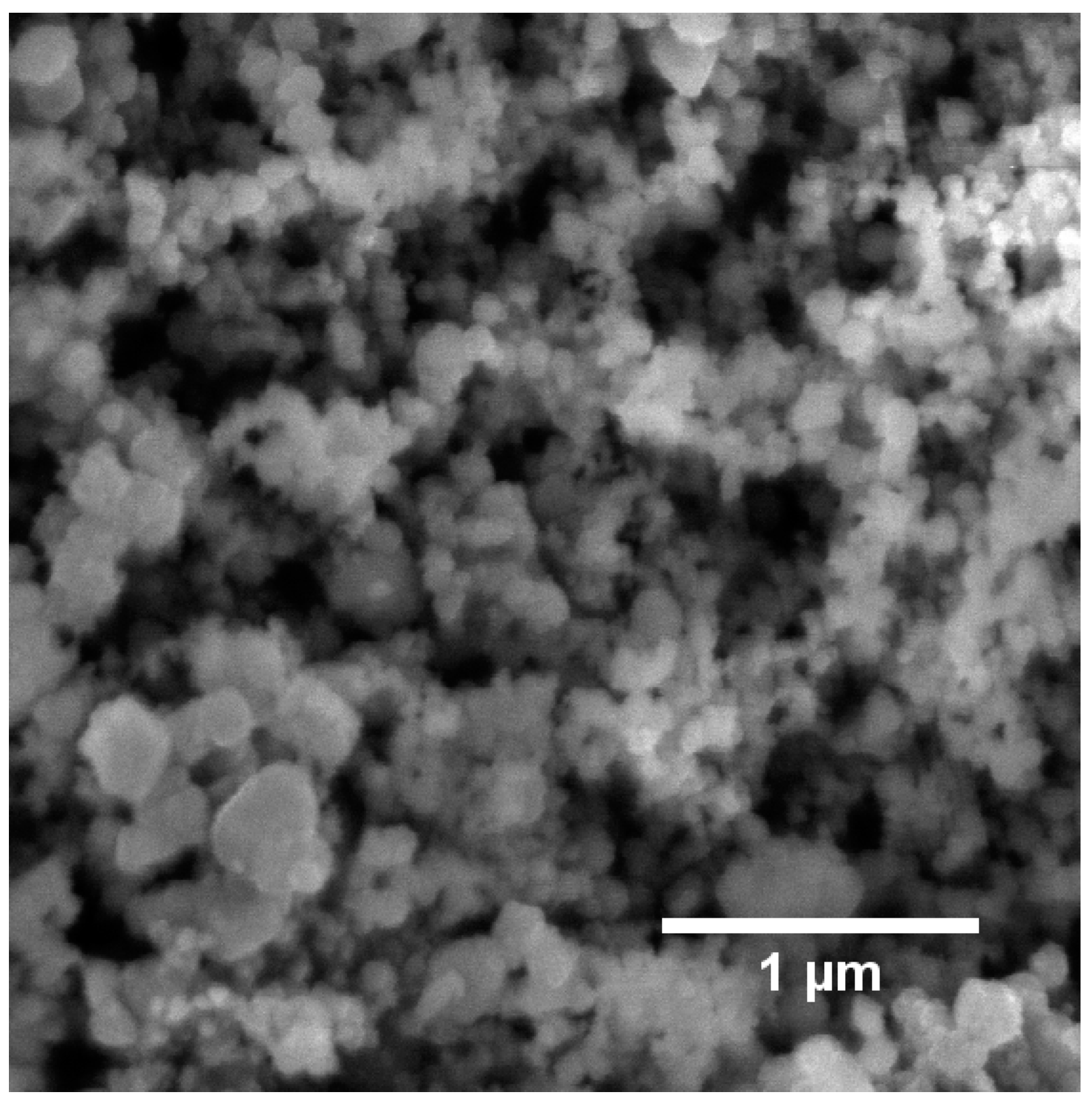This black and white microscopic image showcases a highly magnified view of textured, granular material, resembling a close-up of granite or stone. The image is composed of an intricate pattern of particles that exhibit a range of gray tones from light gray to dark gray, with stark black voids interspersed among them. Small, bubble-like formations are dispersed throughout, adding to the complex visual texture. In the bottom right-hand corner, the image is annotated with a white line above the text "1UM," indicating a measurement scale, further emphasizing the microscopic scale of the material.